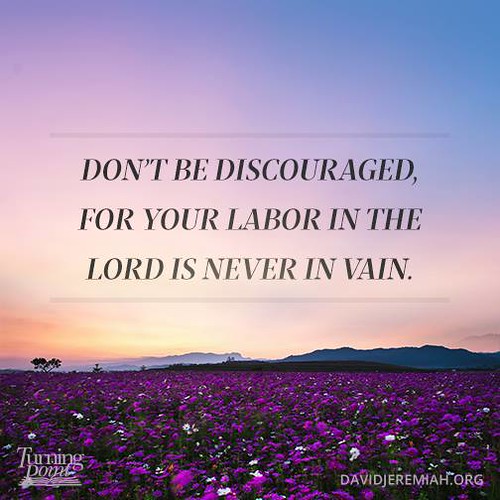In this image, a serene field of vibrant purple flowers dominates the foreground, stretching out towards the horizon where a mountainscape appears in the background, small yet distinct. The sky above is painted with the colors of a sunset, transitioning from pale pink and yellow near the horizon to a dark blue gradient at the top. Amidst this tranquil scene, two or three trees can be seen in the distance, with one larger tree situated off to the left. Text overlays the sky, presented in a black serif font with gray lines above and below, reading, "Don't be discouraged, for your labor in the Lord is never in vain." Additionally, a small logo in the bottom left corner reads "Turning Point," and a URL in the bottom right corner reads "davidjeremiah.org." The image, blending photographic realism and graphic design, conveys a message of encouragement amidst a calm and picturesque natural setting.